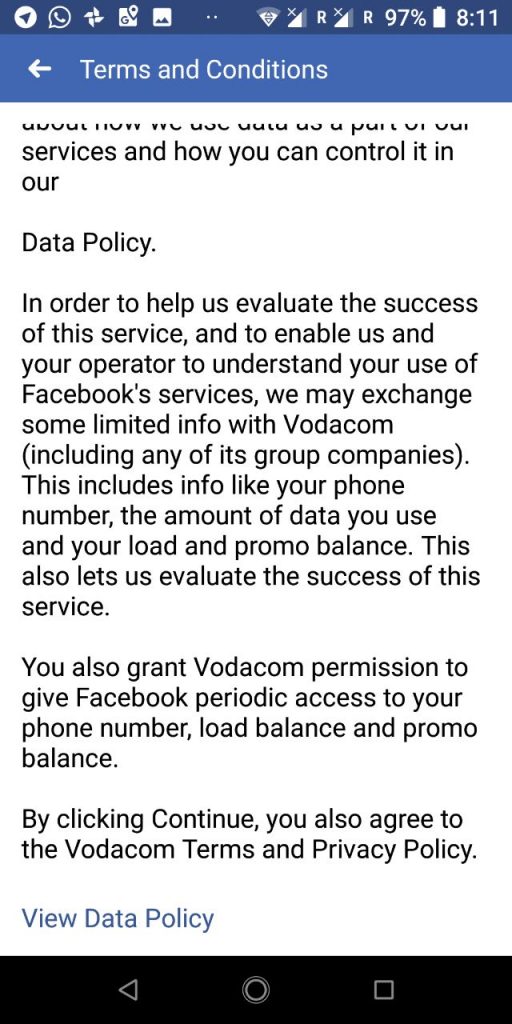This image is a detailed screenshot of a "Terms and Conditions" page taken on an Android mobile phone. The top notification bar is densely populated with various icons, including WhatsApp, Google Photos, Google Maps, and a screenshot icon. The status indicators, such as battery percentage and time, are displayed in white against a dark blue background.

Below the notification bar, there is a blue header displaying the title "Terms and Conditions" in white font. The main page, where the terms are listed, features a white background with black text. The terms outline the services and data policies, describing how the platform, together with the user's mobile operator, Vodacom, may share limited information to understand usage patterns. The details include sharing the user's phone number, data usage, load balance, and promo balance with Facebook. Users are asked to agree to these terms by clicking "Continue" and are provided with a highlighted link labeled "View Data Policy" for more detailed information.

At the bottom of the screen, the black home bar is visible, containing three navigation icons: the Back button, the Home button, and a square button for accessing open tabs on the device.

The screenshot provides a succinct yet thorough preview of the terms users must agree to, with clear visual separation between the notification bar, header, terms content, and navigation bar.